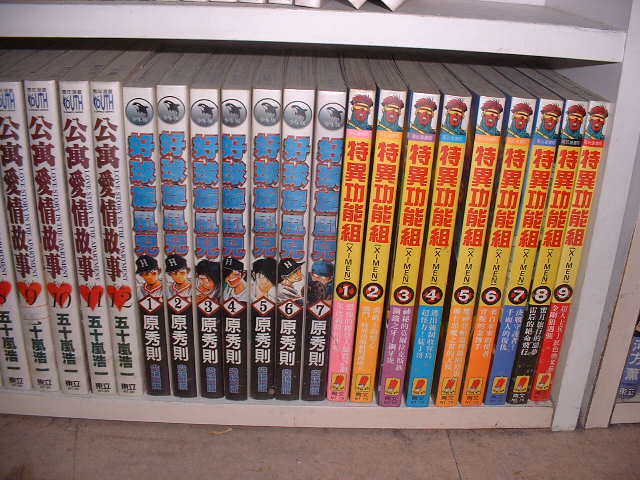The image captures a shelf at floor level, displaying a diverse collection of DVDs with spines primarily labeled in Japanese. The photograph, taken from a kneeling perspective, shows two distinct shelves. The flooring visible is grey tile with subtle marking lines and minor aging in the lower left corner. To the right on the bottom shelf, a series of nine yellow DVDs showcases the X-Men, easily recognizable by the English text and logo. Adjacent, a set of seven white DVDs, possibly depicting characters in baseball uniforms, features a circular emblem which might be a dolphin, and blue text. To the left, a series numbered 8-12 stands out with red heart designs on the spines. The top shelf’s bottom is just visible, hinting at the continuation of the collection but dominated by the focus on the neatly organized lower shelf.